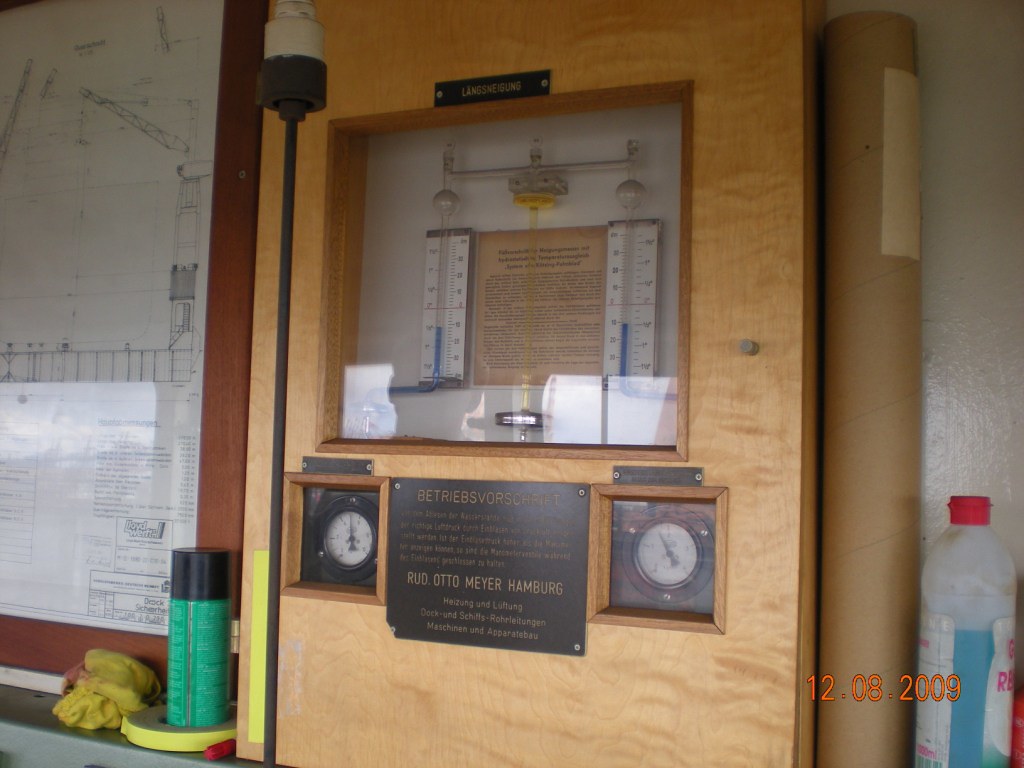This photograph captures an interior scene, possibly taken from inside a science laboratory, classroom, or museum. The centerpiece of the image is a large wooden cutout embedded within a wall. This cutout features a glass window enclosing what appear to be two thermometers. Between the thermometers is an old, tan sheet of paper filled with black text, though the lettering is too small to be legible from this distance.

Below this main glass section are two small clocks, each encased in its own glass window on the left and right sides. Centrally located between these clocks is a rectangular plaque in a blackish-brown color, inscribed with text in German.

Flanking this wooden cutout, on the left side of the image, are several framed blueprints in a wooden frame. Below the blueprints is a can of spray. On the right side, a large cardboard container stands, seemingly designed to store or protect posters. Adjacent to this container is a small bottle. The surrounding environment further hints at the educational or scientific setting with various items and decor typical of a learning or exhibit space.